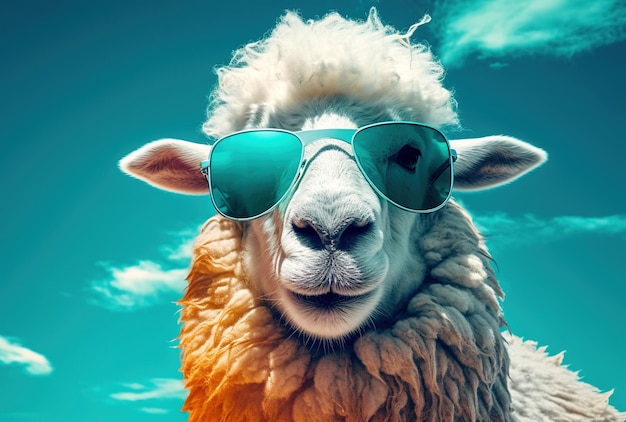This highly detailed, computer-generated graphic art features a close-up of a sheep (possibly confused with a llama) wearing large, silver-rimmed sunglasses. The sheep's face is prominently centered, staring directly at the viewer. The fluffy, curly white hair on its head is adorned with a stringy white part. Its ears stick out sideways, with the left ear pointing left and the right one pointing right. The fur on the left side of its face is a brownish-white color while the fur on the right side has a grayish-white hue. The sheep's thick neck fur appears matted, with the right side showing a whitish beige color and the left displaying an orange tint, likely created by the sun’s effect. The background features a gradient sky, transitioning from a turquoise blue near the sheep to a darker blue towards the top, filled with scattered white, feathery clouds. A subtle green hue emanates around the left lens of its sunglasses, adding an interesting visual element to the overall artwork.